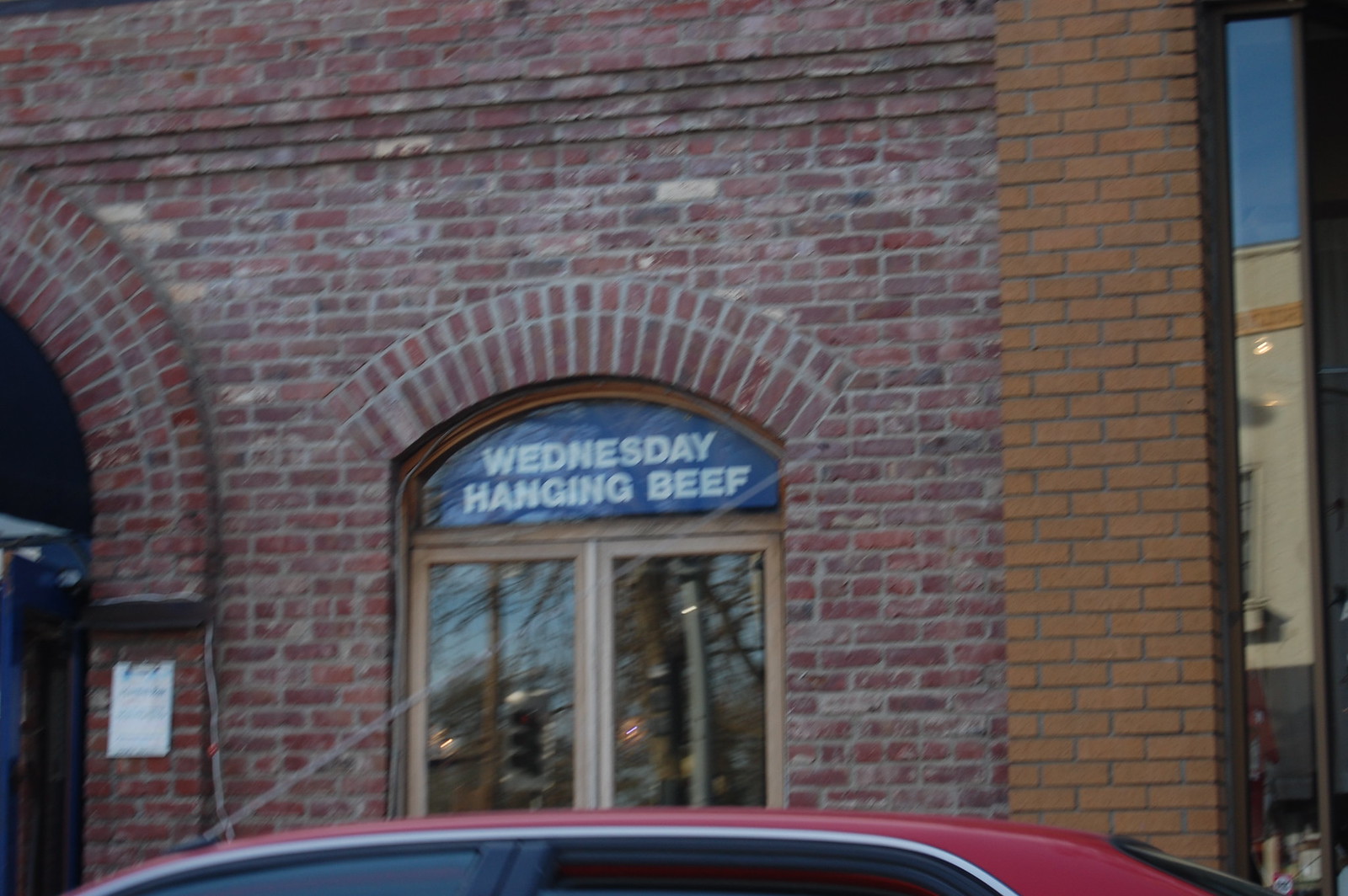This daytime photograph captures the front facade of a red brick building taken from the street. In the foreground, the upper half of a red car parked at the curb is visible, providing a partial frame for the main subject. The building features a central entrance with a set of glass doors flanked by windows and topped with an elegant brick arch. Above the entrance, a blue sign with white lettering prominently displays the words "Wednesday Hanging Beef." The entire composition harmonizes the architectural details with the vibrant elements of the street scene.